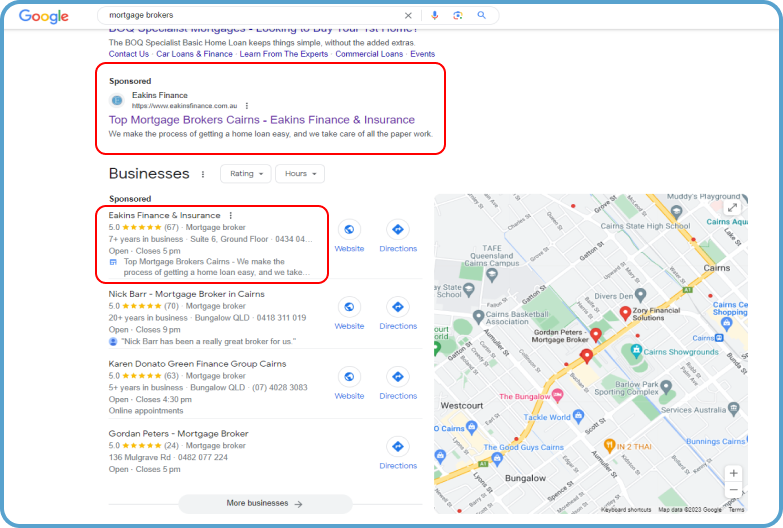The image is a left-to-right horizontal screenshot, likely taken from a computer or smartphone. It features a white background typical of digital screens, encased within an aqua blue border with rounded edges. In the upper left-hand corner, the Google logo is prominently displayed.

At the center of the image, there is a search box containing the query "mortgage brokers," complete with the associated icons: a gray 'X' for clearing the search, a microphone for voice input, and a magnifying glass for initiating the search. 

Below the search box, a sponsored ad for "Eakins Finance and Insurance" is highlighted with a red rounded rectangle. Following this, the word "Businesses" appears in black, indicating the start of organic search results. The ad for "Eakins Finance and Insurance" is repeated with the same red outline.

Further down, additional mortgage brokers are listed, including "Nick Barr Mortgage Broker," "Kevin Donato Green Finance Group," and "Gordon Peters Mortgage Broker." For each entry, options for visiting their website or obtaining directions are available, except for Gordon Peters, which only offers directions.

A gray button labeled "More businesses" is situated at the bottom, inviting users to explore further. On the right side of the image, there is a map indicating the locations of the mentioned mortgage brokers, providing a visual reference for potential clients.